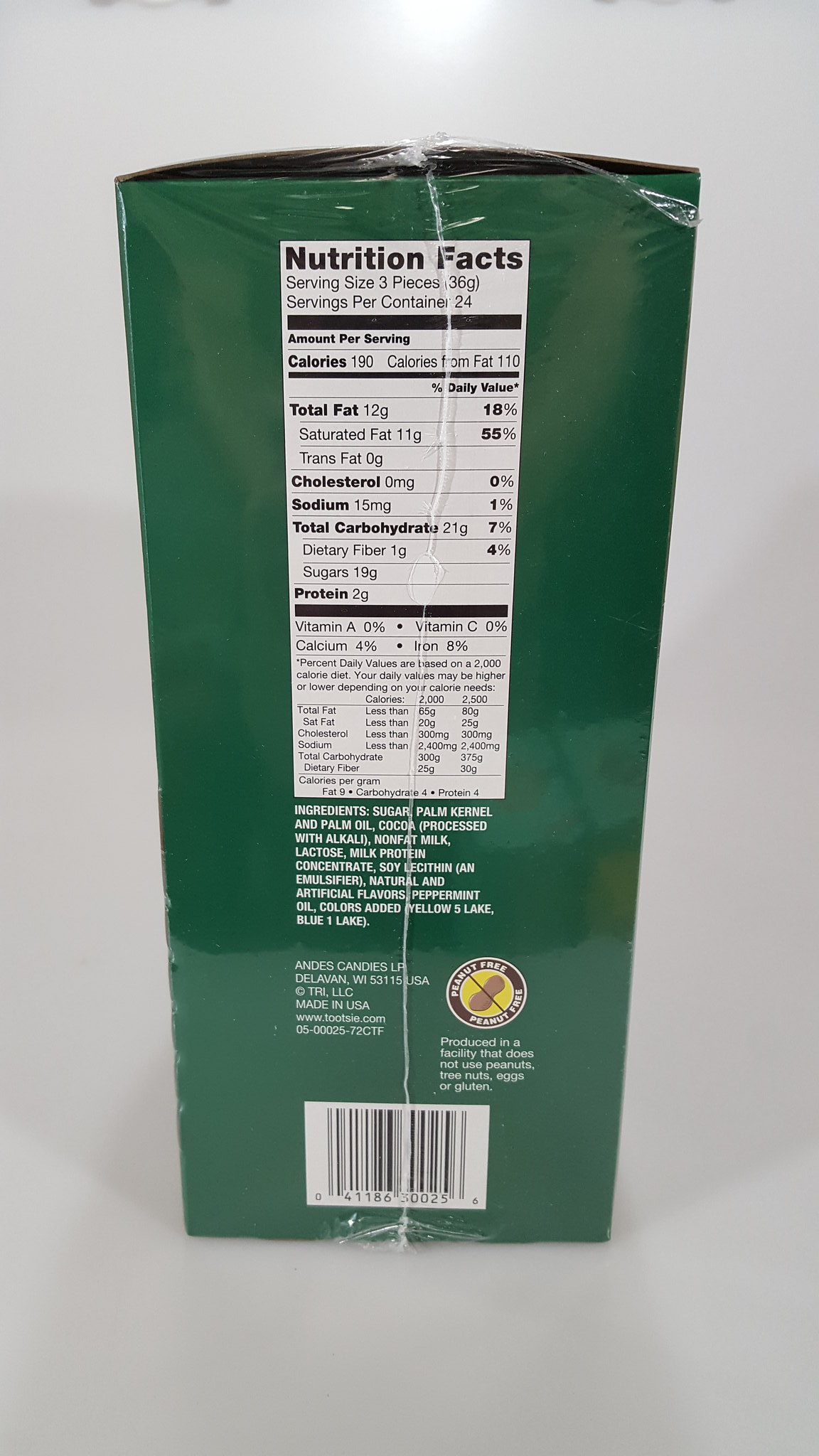The image displays a close-up of a dark green cardboard box, meticulously photographed against a white background, highlighting its product photography quality. The box, still factory-sealed in see-through plastic, is positioned on a white surface where shadows are cast to the left, right, and back. This packaging features a prominent "Peanut Free" label, characterized by a circle containing a yellow background, a brown peanut with a black X through it, and the text "peanut free" repeated around the outer circle.

At the top of one side, the box bears a comprehensive "Nutrition Facts" label in bold black text on a white background. This label indicates the serving size as 3 pieces (36g), with 24 servings per container. Key nutritional information includes 190 calories per serving, 12g total fat (18%), 11g saturated fat (55%), 0g trans fat, 0mg cholesterol, 15mg sodium (1%), 21g total carbohydrates (7%), 1g dietary fiber (4%), 19g sugars, and 2g protein. Vitamin percentages are listed as Vitamin A (0%), Vitamin C (0%), Calcium (4%), and Iron (8%).

Beneath the nutritional information, there's a detailed list of ingredients: sugar, palm kernel and palm oil, coconut processed with alkali, nonfat milk, lactose, milk protein concentrate, soy lecithin (an emulsifier), natural and artificial flavors, peppermint oil, and added colors such as Yellow 5 Lake and Blue 1 Lake.

Towards the bottom of the box, it lists the manufacturer as "Andes Candies," specifying the address: 53115 Delavan, Wisconsin, USA. The packaging also highlights that the product is made in a facility that does not use peanuts or tree nuts. Additionally, there's a barcode centered at the bottom, alongside the manufacturer's website details.

The photograph captures the meticulous packaging and labeling of the product, reflecting its detailed presentation and adherence to allergen safety.